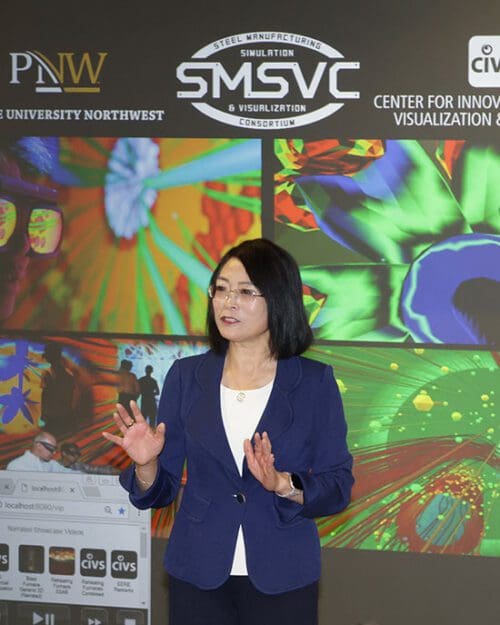The photograph captures an Asian woman of mature age, with short, shoulder-length, straight black hair parted at the center, giving a dynamic speech on stage. She's wearing thin wire-rimmed glasses that subtly indent her face, a blue blazer with a single button over a white crew-neck shirt, a necklace, and black slacks. Her expressive posture includes her arms bent at the elbows with her palms facing up, as if she's in the midst of a passionate explanation. Behind her, a large projection screen displays vibrant and colorful images in four panels. Accompanying text on the screen reads "PNW University Northwest," "Steel Manufacturing Simulation, SMSVC," and "Center for Innovation Visualization," indicating that her lecture is likely focused on simulation and visualization topics related to innovative manufacturing techniques.